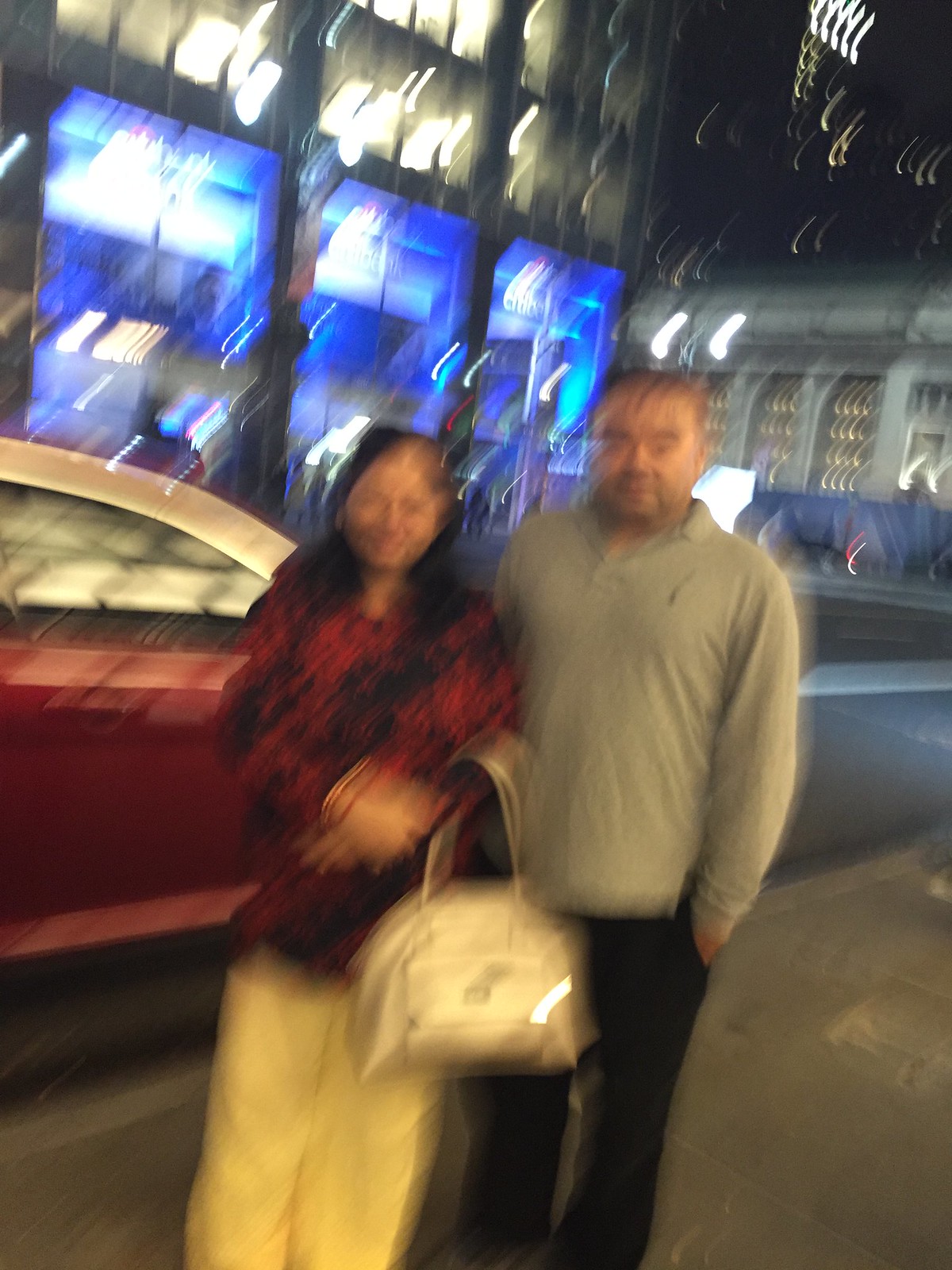This low-resolution, motion-blurred image captures a moment outdoors, featuring two individuals standing side by side. A woman positioned on the left has black hair and is dressed in a black and red top, complemented by black pants. She is holding a white bag on her left arm. To her right stands a man dressed in a gray sweater and black pants. Behind them, toward the left side of the image, a red car is faintly visible.